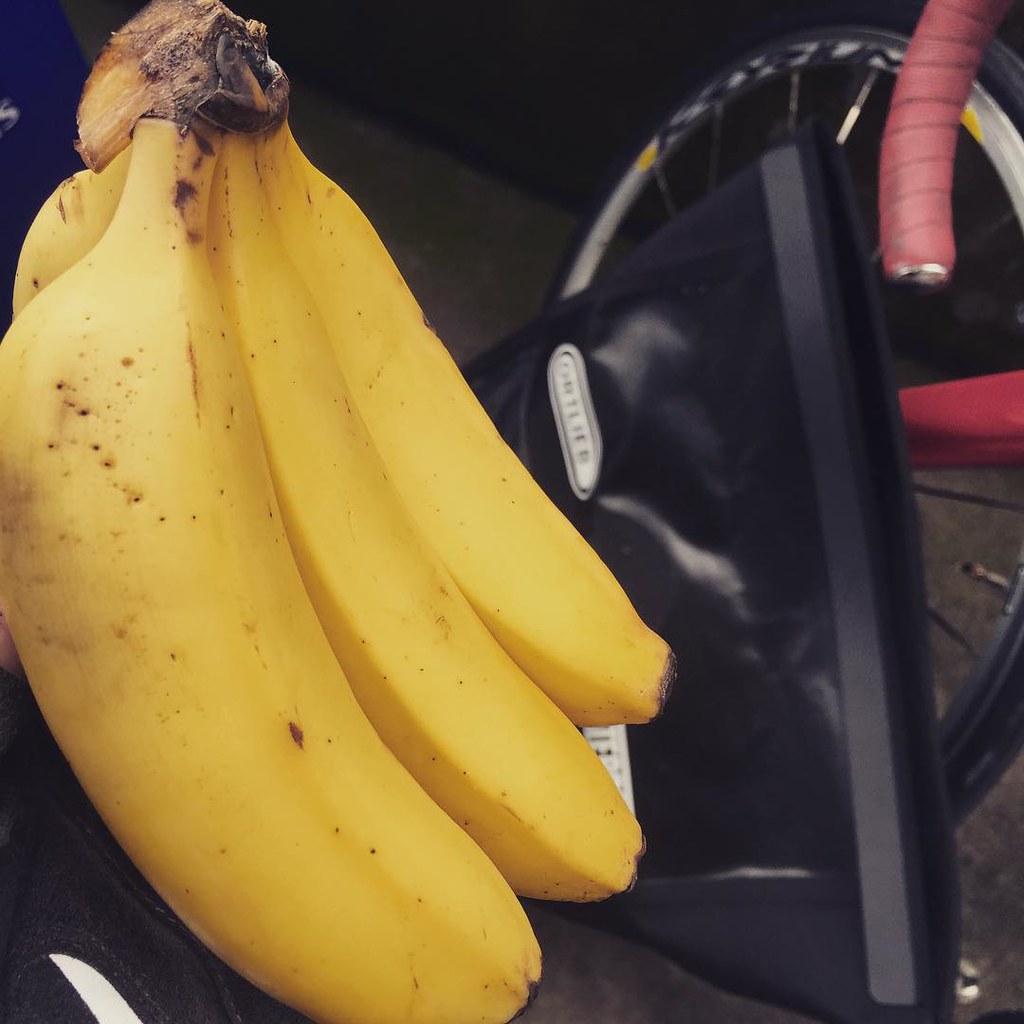This photograph captures a bunch of thick yellow bananas, just about ripe with a few brown spots scattered across their skins. The cluster, consisting of at least four, potentially five bananas, lies prominently in the left foreground. One of the bananas, in particular, stands out due to its unusual girth. Adjacent to the bananas is a bicycle, characterized by its red frame and orange-taped handlebars. The front wheel of the bike is clearly visible with a black tire. To the right of the bananas and partly obscuring the bicycle, a black shiny bag with unreadable text and a central zipper can be seen. Something blue with the letter 'S' is situated behind the bananas, adding a pop of color against the brown, speckled surface that suggests a dirty floor. In the background, a black object aligns with the wall, adding depth to the scene.